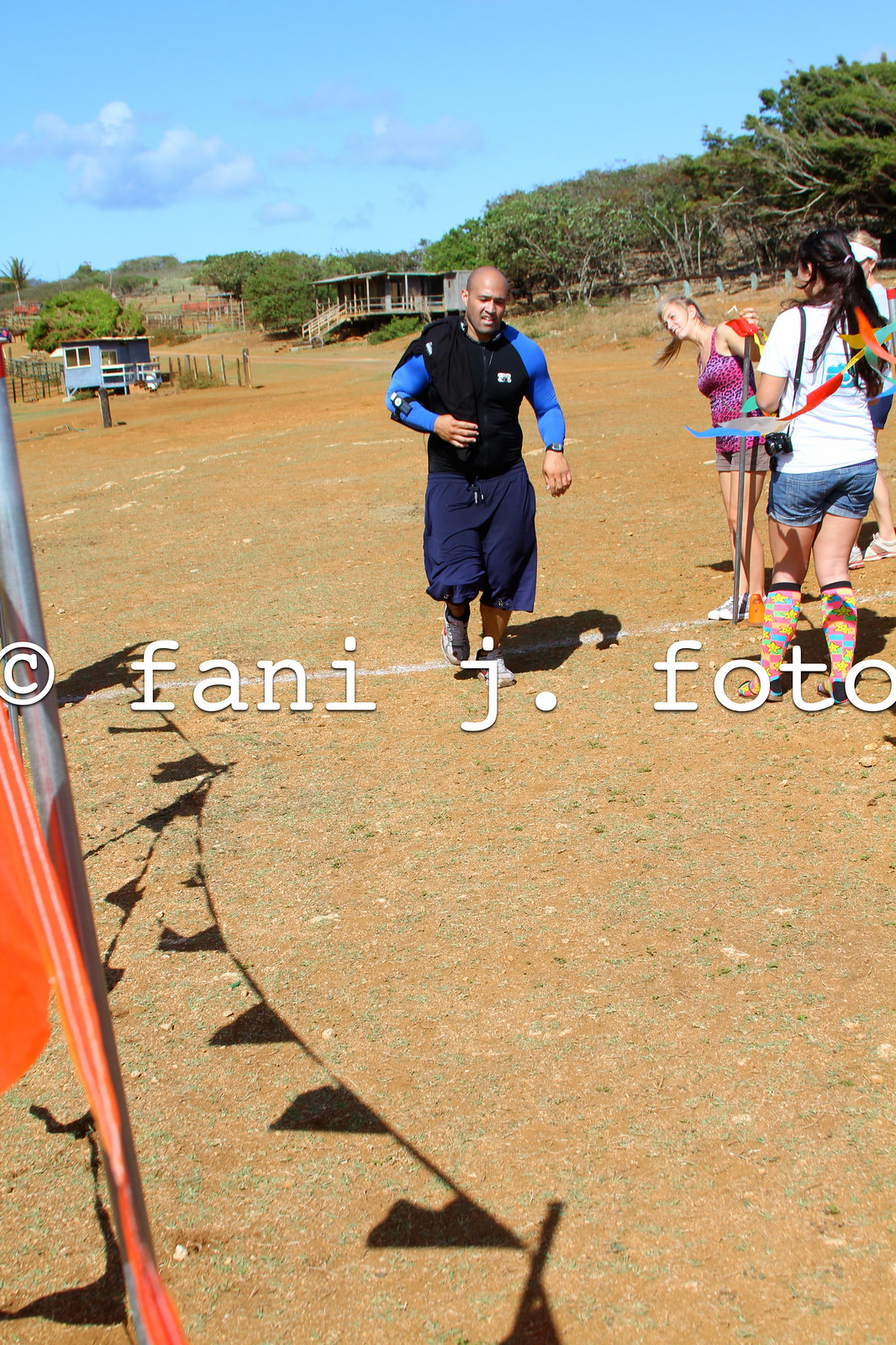In a tropical, impoverished area under a clear blue sky dotted with light clouds, a dirt landscape sparsely patched with dying grass stretches out. In the foreground, a bald South Asian man, mid-jog with a pained expression, is dressed in a black vest with a white splotch, an aqua blue shirt, and navy blue shorts, while an MP3 player is strapped to his arm. To his right, a smiling Caucasian woman in a purple leopard-print tank top, and another woman in denim shorts and a white shirt with colorful puzzle-piece socks, stand in casual conversation. In the background, poorly constructed wooden shacks and a mix of trees, including a barely discernible palm tree, add to the scene's rustic charm. Shadows of a line of flags, possibly orange, are cast on the ground, hinting at festive or demarcating banners overhead. Right across the middle of the image, the copyright text reads "Fanny J. Photo," spelled "F-O-T-O," marking the photograph.